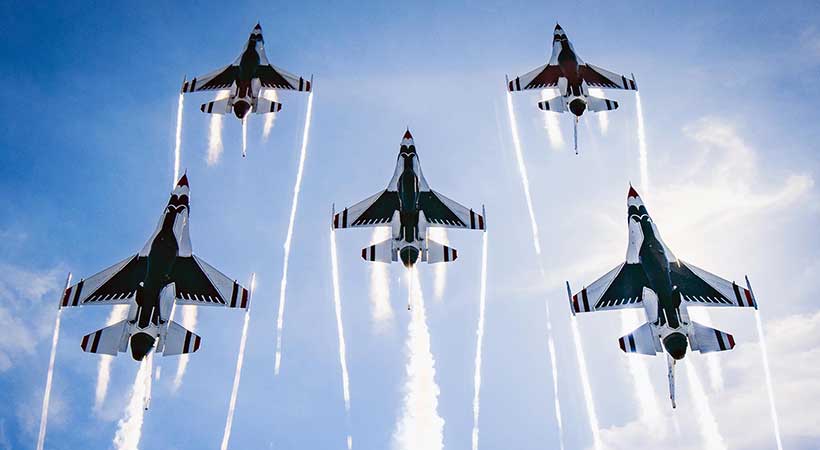The image captures a striking scene of five fighter jets, each sleek in silver and black, soaring upwards through a bright blue sky streaked with sparse clouds. The jets are arranged in a tight, precise formation: two leading at the top, one centrally placed, and two following at the back. Each aircraft features distinctive hawk insignias and are equipped with sharp, pointed noses, large front wings, and smaller rear wings. As they ascend, they leave trails of white smoke plumes, creating dramatic lines in the sky. The sun peeks from behind the clouds, illuminating the upward momentum and the powerful unity of the jets in motion.